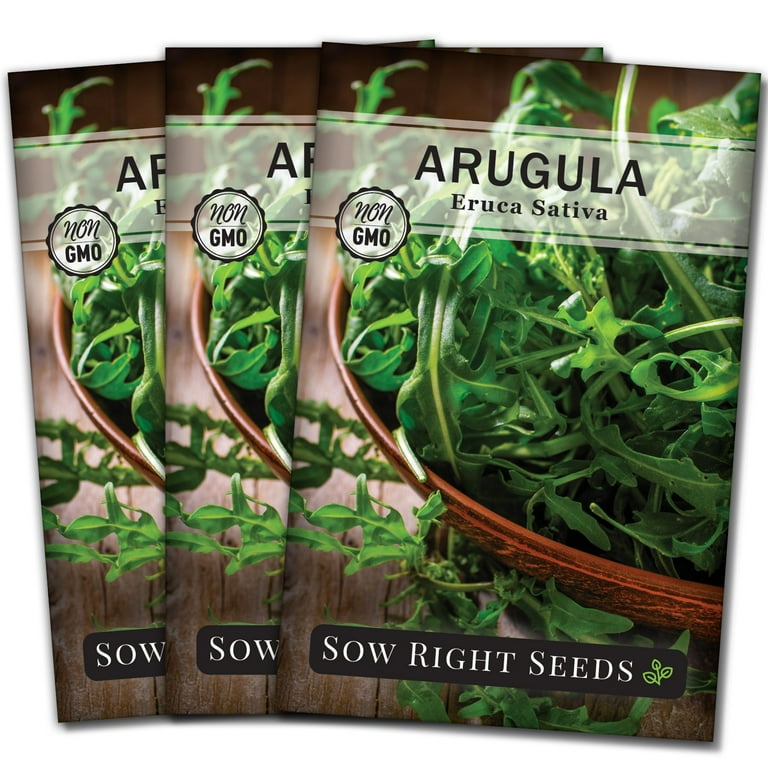This image features three identical packets of arugula seeds from Sow Right Seeds. Each packet showcases a rustic design with a backdrop resembling reclaimed wood. Dominating the front is a bowl of freshly harvested arugula, presented in a brown earthenware crock bowl, with additional arugula leaves scattered on the wooden surface. The top of each packet displays the word "Arugula" in bold, accompanied by its botanical name, "Eruca Sativa," and a "Non-GMO" label in the upper-left corner. The brand name, "Sow Right Seeds," is prominently featured at the bottom, alongside a logo depicting three leafy stems. The packets incorporate a color palette of brown, silver, black, green, and white, with text elements in brown, adhering to the earthy and natural aesthetic.